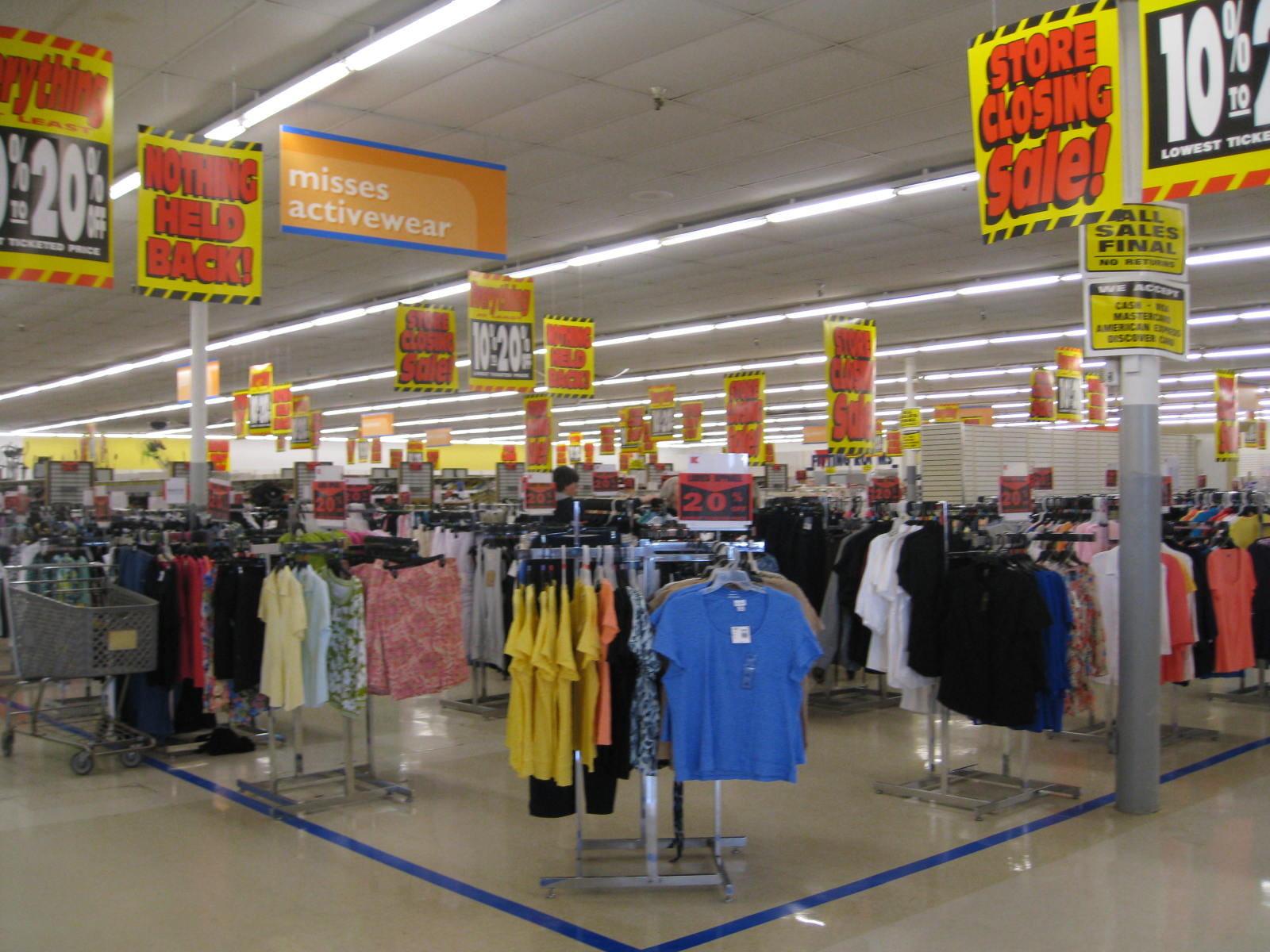This detailed photograph captures the interior of a department store during a store closing sale in the Mrs. Activewear section. The store's layout includes a shiny, light beige linoleum floor with a blue border delineating the area filled with racks of various clothing items. The ceiling is composed of rectangular, drop ceiling tiles interspersed with bright white, fluorescent cylinder lights arranged in neat rows.

Dominating the center of the image is a freestanding, four-section metal rack prominently displaying blue t-shirts. Surrounding this are additional racks showcasing a variety of garments, including yellow blouses, pink and light yellow skirts, black, white, and peach blouses, and assorted button-up shirts with different neck styles. A shopping cart is positioned on the left side, adjacent to one of the clothing racks.

Throughout the space, a collection of signs hangs from the ceiling, announcing details of the ongoing sale. These signs declare significant discounts, ranging from 10% to 20% off, with phrases such as "store closing sale," "nothing held back," "all sales final," and specific payment options accepted, including cash, MasterCard, American Express, and Discover. The coordinated arrangement and diverse assortment of clothing items reflect the systematic yet bustling atmosphere typical of a store in its final days of operation.